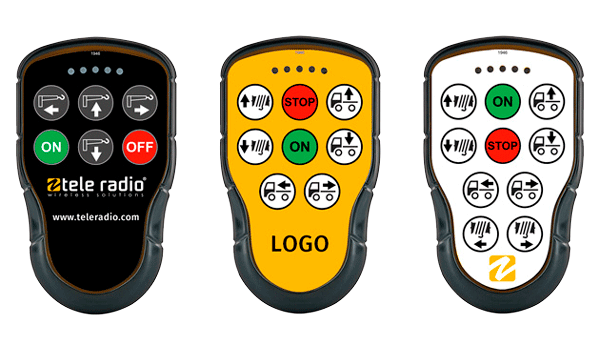The image displays three handheld controllers against a white background, arranged horizontally in a row. All three devices share a similar shape: rectangular and vertical, with slightly curved inward sides leading to an oval bottom. Each controller features different button configurations and face designs.

The controller on the left is a dark gray color with a black interior. It has a total of six buttons, organized in two rows of three. At the bottom row, a green "on" button is on the left, and a red "off" button is on the right. Below the buttons, the text "Teleradio" and the URL "www.teleradio.com" are visible.

The middle controller has a yellow interior with a black border and is equipped with eight buttons, arranged in three rows of three at the top and middle, and two on the bottom. In the center are a "stop" button and an "on" button. The word "logo" appears at the bottom.

The rightmost controller is white with a black border and contains ten buttons, distributed across four rows: three on the top, three on the second, two on the third, and two on the fourth rows. This one also features an "on" button and a "stop" button in its center. At the bottom, there is a logo consisting of an orange square with a white zigzag.

Each controller appears to be designed for operating machinery, possibly cranes or truck-mounted equipment, indicating their robust and functional design for industrial use.